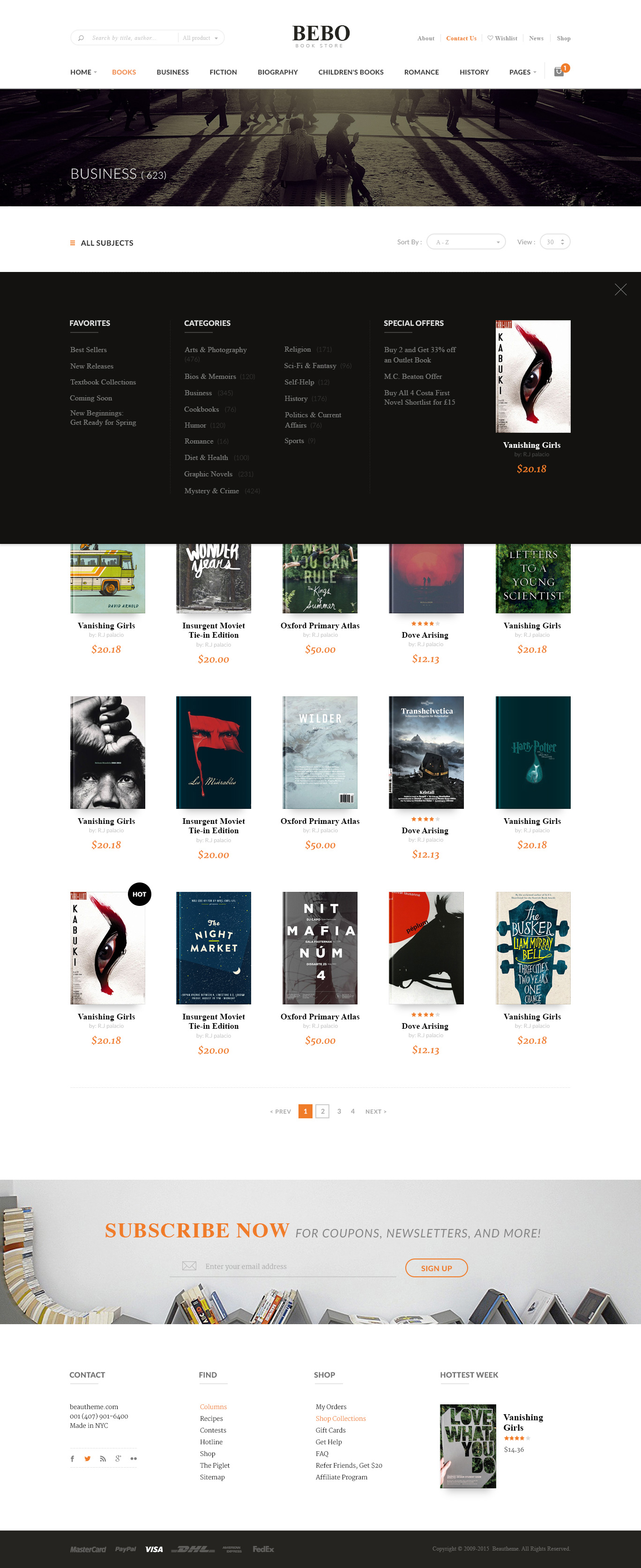The website, which seems challenging to read, is branded with "Bebo" at the top. To the left, there is an apparent search box, while to the right, some menu items are indiscernible. Directly below the top section, there is a horizontal navigation menu in black lettering with eight unreadable categories. 

Beneath this menu, a rectangular image shaded in black and grey displays a group of people, with the word "Business" positioned in the lower-left corner. Further down, a larger rectangular section contains another set of menu items and features a layout divided into four columns, each with an associated image, though the text here is hardly legible due to its small font size.

Lower on the page, there are rows of book covers, organized into five books per row over what appears to be three rows, with text descriptions that are unfortunately unreadable. Just below this book section, there’s a page counter equipped with arrows for navigating through different pages.

Further down, a subscription box encourages visitors to "Subscribe Now" for coupons, newsletters, and more. The very bottom section of the website lists additional categories like "Contact," "Fax," and "Shop," each with various subheadings that are not specified.